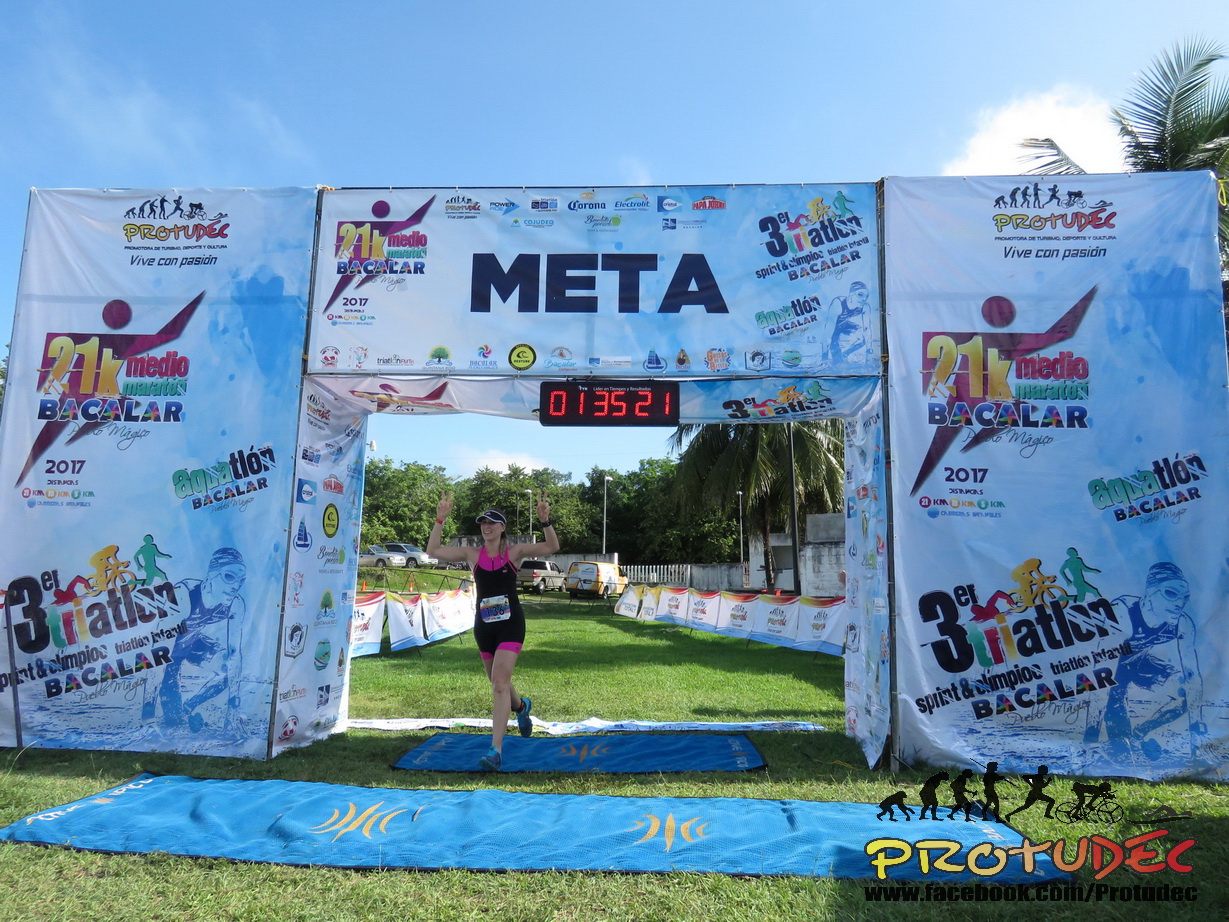The image captures a vibrant moment in a 21k marathon held in 2017, marked by a prominent META banner at the finish line. The elaborate, temporary white gate is adorned with sponsor advertisements, including a logo that appears to say PROTUDEC. Dominant under the center of the META banner is a large digital timer displaying "01:35:21." Beneath this structure, a jubilant woman in pink and black running apparel, including a visor and blue sneakers, crosses the finish line. She raises both arms in celebration, making peace signs with her hands and beaming with a triumphant smile. She is the sole runner visible in the photograph, adding a sense of solitary achievement to the captured moment. The backdrop includes some cars and grassy terrain, emphasizing the organized yet temporary nature of the marathon setup.